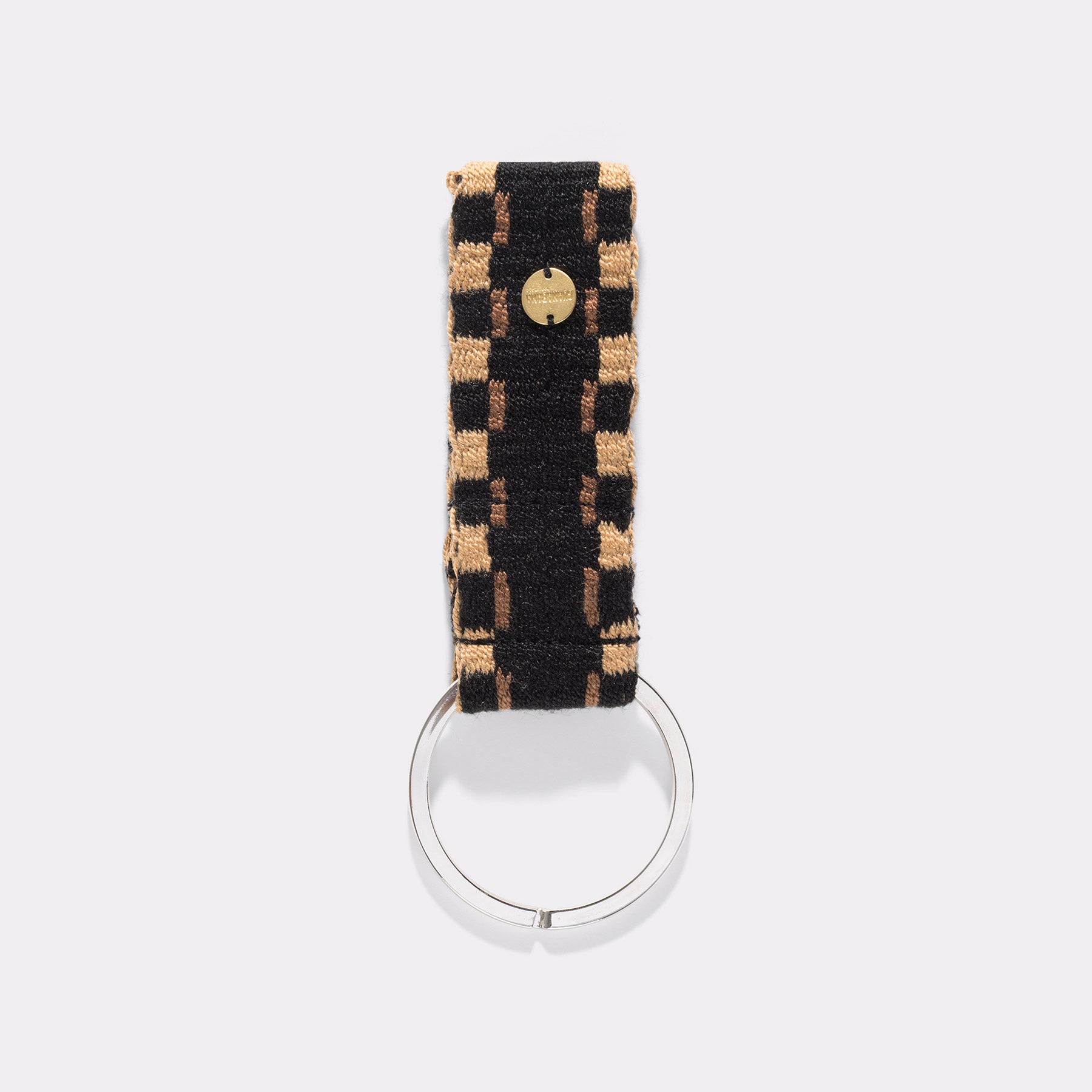Displayed against a solid white background, the close-up image features a keychain without any attached keys. At the bottom of the keychain is a transparent acrylic loop designed to hold keys. Above this loop, a silver metal ring provides additional attachment points. The central segment of the keychain is a vertically oriented rectangular fabric piece showcasing intricate woven stitching. This woven fabric has a distinctive pattern: a dark brown stripe runs vertically down the middle, flanked by a crisscross checkerboard design of dark brown and light tan squares. Amidst the checkerboard pattern lies a circular gold-colored maker's mark, adding a touch of embellishment to the overall design.